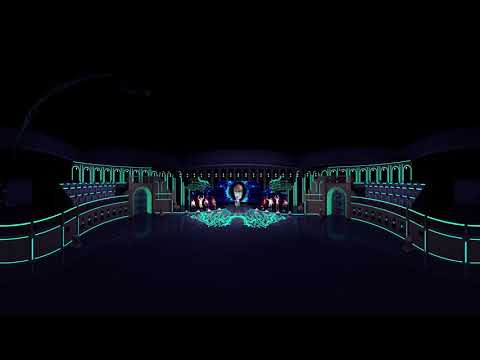The image depicts a night scene at an outdoor theater or stadium, characterized by a detailed and almost surreal quality, possibly resembling a drawing. To the left and right sides of the image, there is turquoise fencing with gray accents. Centrally, we see a turquoise grouping that resembles an audience, though the detail is minimal. A stage dominates the center of the composition, featuring seven performers who might be actors, standing on the left and right sides. The center of the stage is occupied by a large blue area, possibly depicting a photo or projection of a person with reddish hair, seemingly holding their arms out to the sides. Above this stage, you can see lighting fixtures. On either side of the stage, there are structures reminiscent of a Greek temple, adding to the theatrical ambiance. The top half of the photo is enveloped in a dark, black sky tinged with purple hues, either from artistic coloring or subtle lighting. The overall scene is bathed in neon or ultraviolet luminescent paint, giving the impression of glowing in the dark, contributing to the ethereal and vibrant atmosphere.